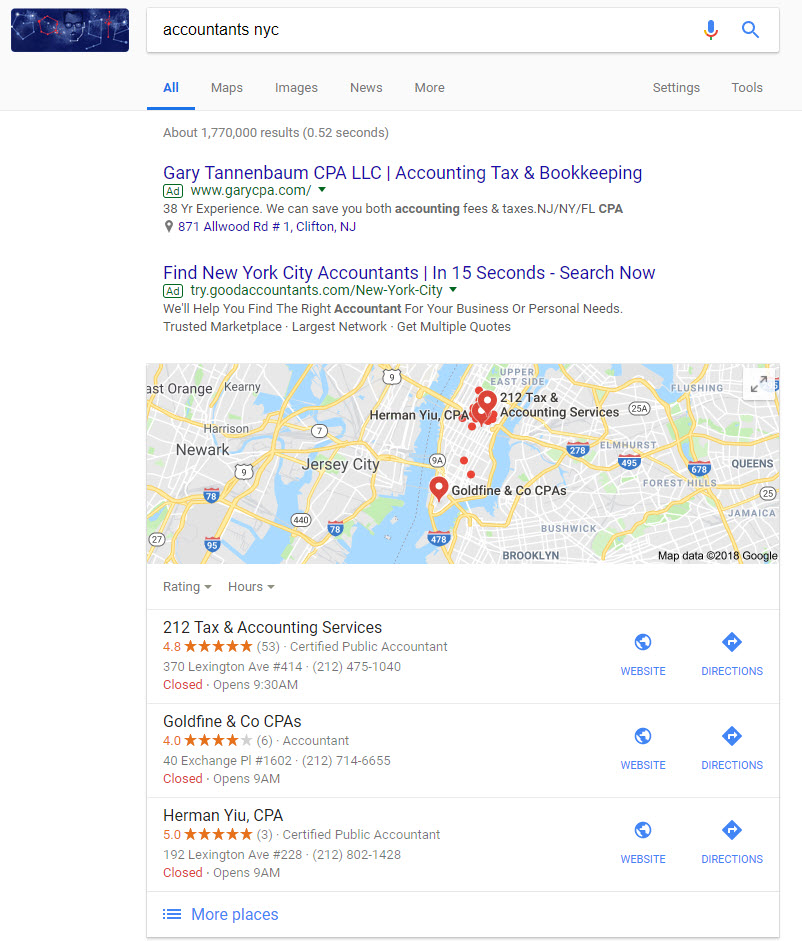The screenshot displays a Google search for "accountants in New York City." At the top of the image is the search box with the query. Below it, several tabs are visible: "All" is highlighted in blue and underlined, and the sub-tabs "Maps," "Images," "News," and "More" are in gray. Further to the right is "Tools" in gray. The search results indicate approximately 1,770,000 results returned in 0.52 seconds.

The first search result features Gary Tatenbaum, CPA, LLC. The listing includes keywords such as "Accountant," "Tax," and "Bookkeeping." An ad tag in green is displayed next to the URL "www.garycpa.com." The description highlights 38 years of experience, promising savings on account fees and taxes, with service areas including New Jersey and New York. The address listed is "87 Alleywood Road, #1, Clifton, New Jersey" in blue, indicating it as a clickable link.

A map is present, featuring labeled areas around New York City, including Newark, Jersey City, Brooklyn, Elmhurst, Flushing in Queens, Jamaica, and Rayton.

Additional results visible include:
- 212 Account Services in dark gray,
- Go Find and Co. CPAs,
- Herman UYIU, CPA.

The map on the right likely marks various CPA locations in and around New York City.